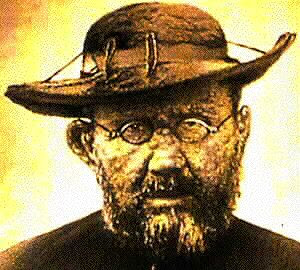The image is an evocative representation of a scruffy, backwoods preacher or an Amish-like figure. It appears to be a deliberately aged photograph, possibly from a movie or television show, with a vintage aesthetic accentuated by yellow and brown tones. The portrait focuses on the man's chest up, revealing his distinctive features: a textured, bumpy face with numerous boils and welts, particularly noticeable on his right ear. He wears a wide-brimmed, dark-colored hat with a strap or belt around it, along with very small round glasses. His facial hair includes both a beard and mustache, enhancing his rugged appearance. The background is a mix of overexposed yellow and white, with a hint of orange in the top left corner, giving the image an eerie, almost surreal quality.